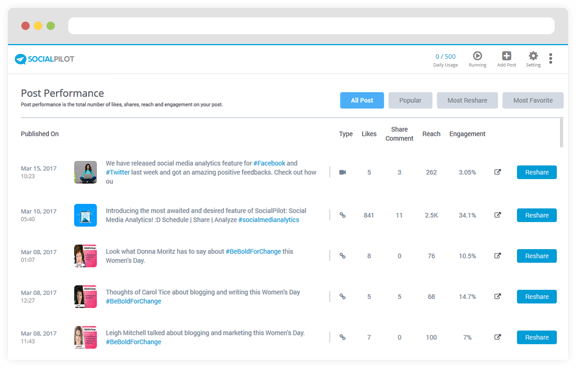The image displays a screenshot from the social media management tool, Social Pilot, as seen on macOS. The interface is sleek and minimalistic, featuring an address bar at the top. The image focuses on the "Post Performance" section for March 2017, which details metrics such as likes, shares, reach, and engagement for various social media posts.

Highlighted within the screenshot, the post that garnered significant attention is titled “Introducing the most awaited and desired feature of Social Pilot – Social Media Analytics.” This post achieved 841 likes, 11 comments, and a reach of 2,500, resulting in an impressive 34.1% engagement rate. Other posts include mentions of notable figures such as Donna Moritz and Carol Tice, discussing their thoughts on blogging, though they received considerably less engagement.

To the right of each post, there are blue 're-share' buttons, enabling users to easily share these posts again. One notable post announced, “We have released the social media analytics feature for Facebook and Twitter last week and got amazing feedback.” This post, however, did not achieve the level of engagement seen with the analytics feature announcement.

Overall, the image provides a comprehensive look at how different posts performed during the specified time period, emphasizing the strong reception of the new analytics feature.